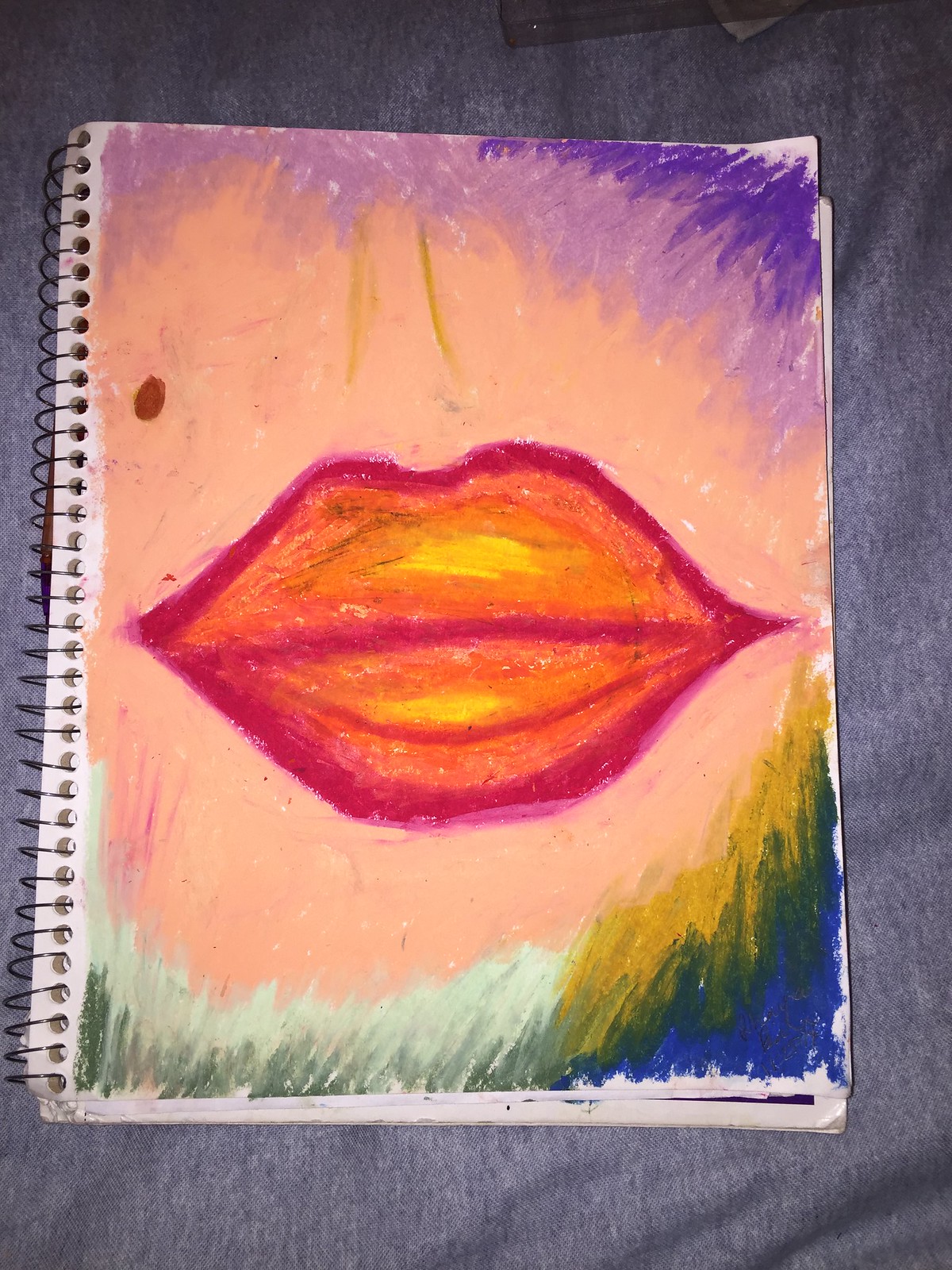This is a photograph of a colorful drawing in a spiral notebook, laying on a gray blanket. The drawing appears to be a watercolor or crayon illustration, possibly created by a student. It features a close-up of the bottom portion of a person's face, focusing on the lips and a hint of the nose above. The nose is represented by two simple yellow lines, while a prominent freckle or mole is visible above the upper lip. The lips are exaggerated in size, outlined in red with vibrant hues of orange, yellow, and red resembling the colors of fire. The face itself has a pale complexion. The top section of the drawing transitions from light to dark purple in a gradient, while the bottom is adorned with a mix of light and dark greens, yellow, and blue. The spiral binding of the notebook is noticeable on the left edge of the image.